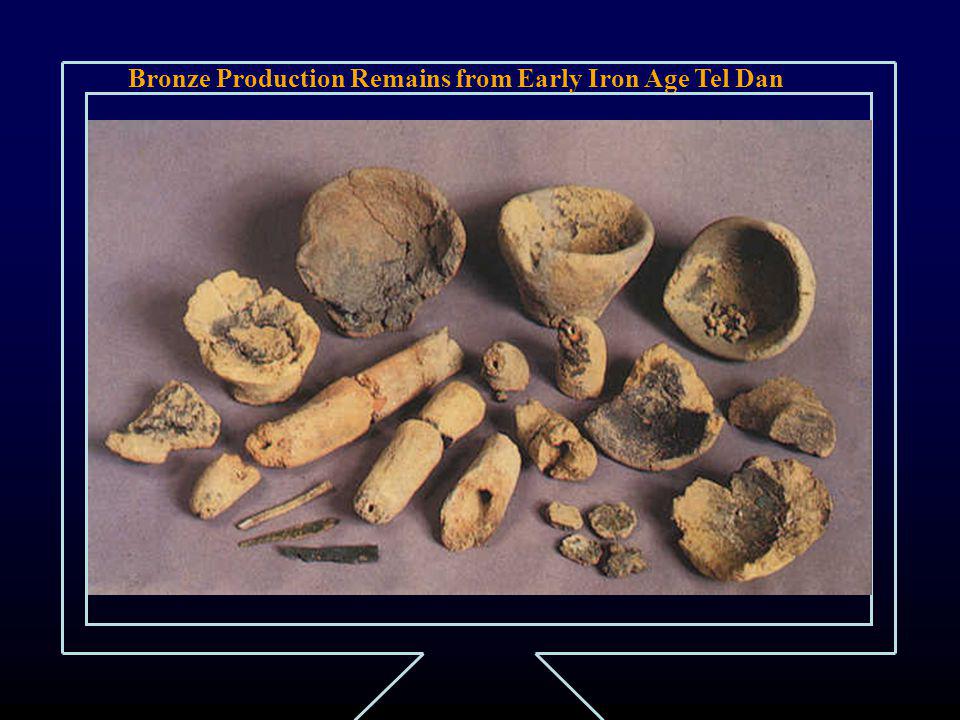The image features assorted archaeological finds identified as "bronze production remains from early Iron Age Tel Dan," written in a brownish, Times New Roman font at the top. The border surrounding the image transitions from royal blue at the top to black at the bottom, resembling the appearance of a TV screen on a stand. The central photograph displays a collection of gray and tan artifacts, including several broken pottery pieces and hollow cylindrical objects. Additionally, there are four small, roundish shards scattered among them. These items, which appear to be weathered and covered in dirt or clay, rest on a plain, matte brown background. The entire composition is encapsulated by white lines that frame both the title and the image itself.